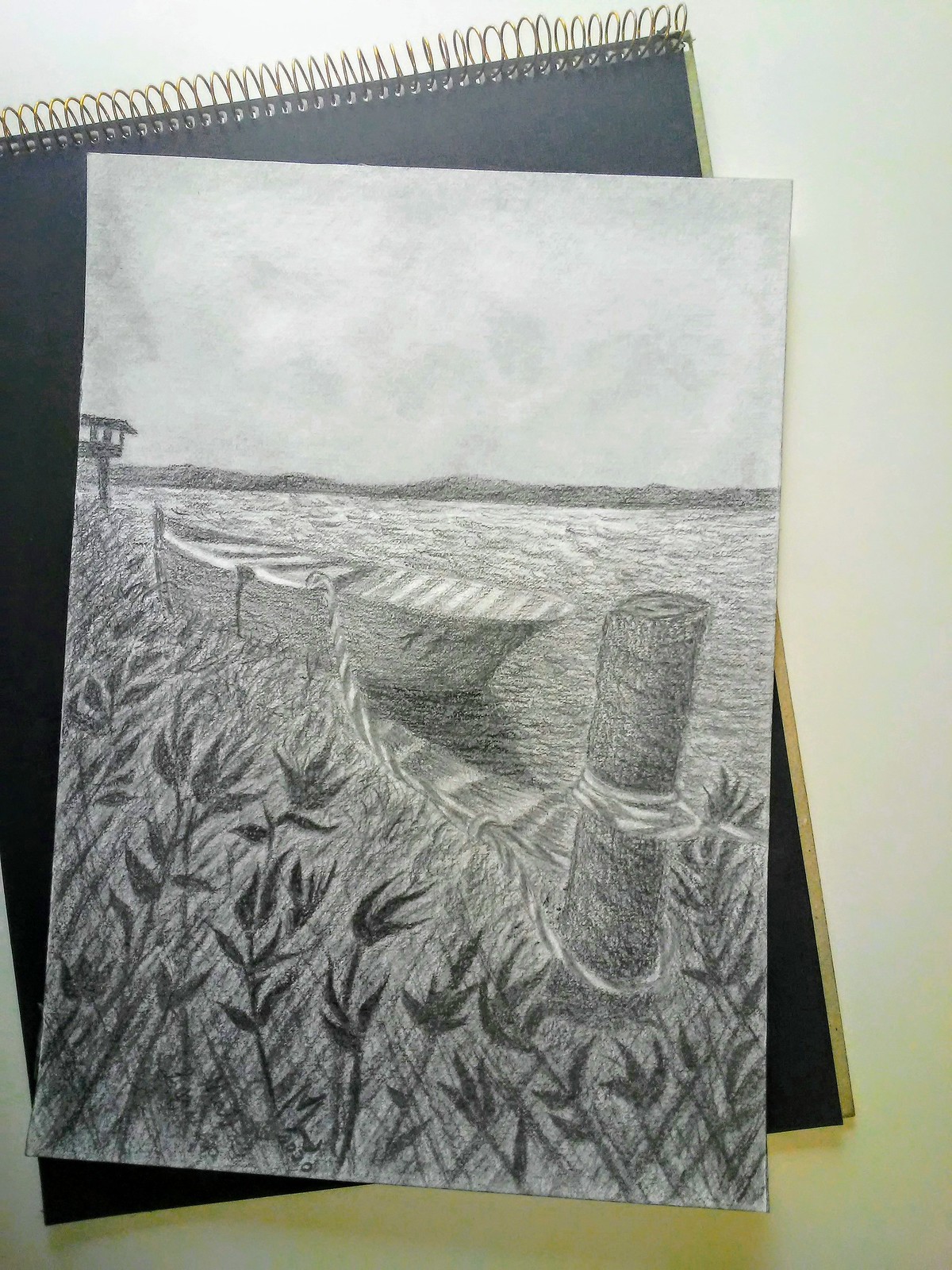This image captures a detailed pencil sketch displayed on a piece of paper that appears to have been torn from a book. The paper is placed atop a black sketch pad with metal spiral binding at the top, all situated on a white surface. The sketch vividly depicts a tranquil lakeside or riverside scene. Central to the image is a rowboat, deeper than an average one, tied to a post with a rope. The boat is positioned along the bank, which is lush with grass and wildflowers. In the background, hills rise gently under a cloudy sky, and small waves ripple across the water. To the left, part of a pier is visible, adding depth to the serene landscape. The entire scene is rendered in pencil, giving it a monochromatic and timeless quality.